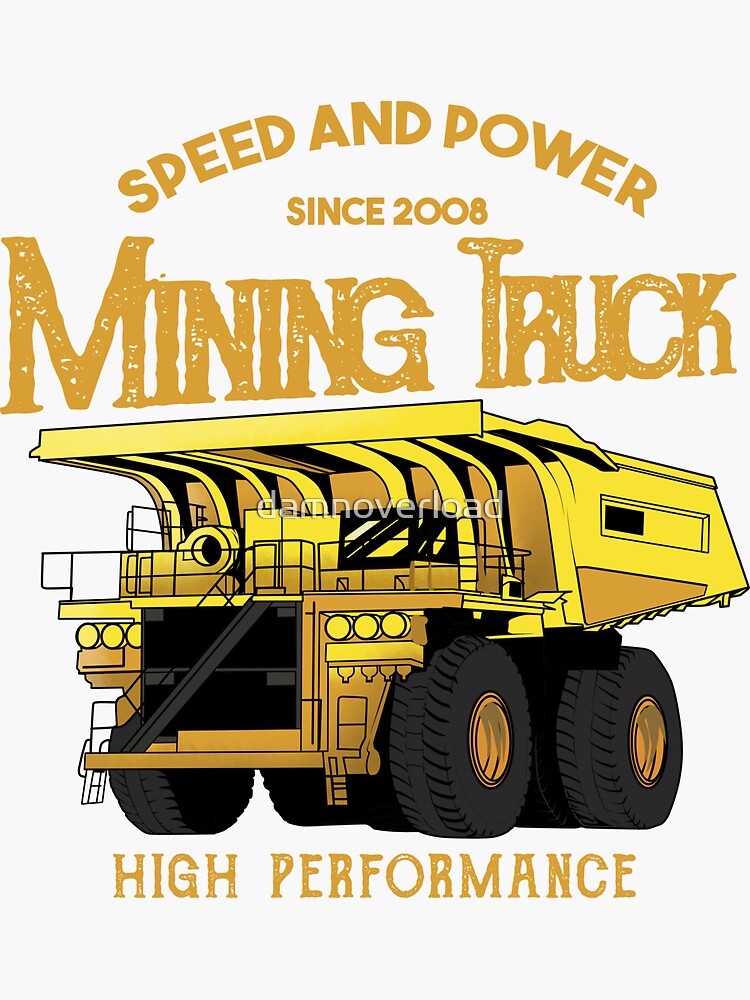The central image features a detailed graphic representation of a large, heavy-duty mining truck rendered in a striking shade of yellow-gold. The truck is prominently placed in the center, showcasing its massive size with four monster wheels—two visible on each side. It has a distinctive design with three headlamps on each side of a black central grille. Above the truck, bold brown text reads "Speed and Power Since 2008, Mining Truck," highlighting its long-standing efficiency. Below the truck, the text "High Performance" is also written in brown. The image is watermarked with the text "Dam Novalode," indicating its source or creator. Overall, the graphic exudes a sense of power and durability, emphasizing its high-performance capabilities.